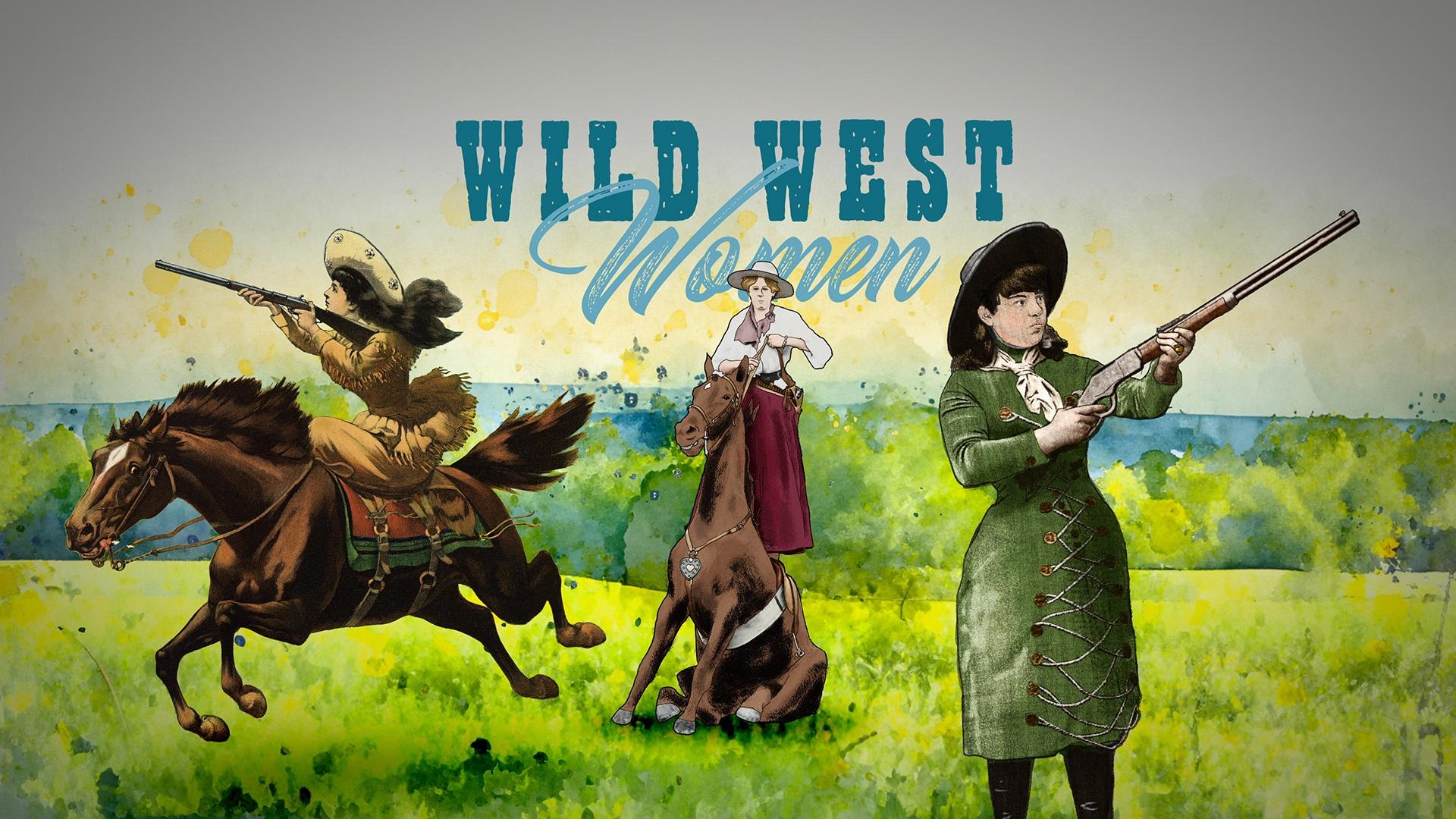The illustration, titled "Wild West Women," appears to be part of an infographic, website, or museum exhibit, featuring bold, teal text at the top. The words "Wild West" are styled in dark teal, cursive or print font, while "Women" is in a lighter teal, italicized font. The scene is set in a grassy green meadow with mountains and a gray sky in the background.

On the left, a woman with long black hair flows behind her as she rides a galloping brown horse side-saddle. She wears a brown suede outfit with fringes, a large brown cowboy hat, and points a rifle towards the left.

In the center, another woman stands firmly on the back of a seated brown horse. She is dressed in a long maroon skirt, white blouse, and pink neckerchief, complemented by a large white hat. At her hip, she carries a holstered pistol.

On the right, a woman in the foreground wears a green, lace-up dress with a white neckerchief and a large black hat. She holds a rifle aimed to the right, displaying a serious expression.

All three women sport period-appropriate cowboy attire, conjuring an 1800s Wild West ambiance, reminiscent of iconic figures like Annie Oakley. The painting's style is somewhat cartoonish, yet rich in dynamic action, showcasing the strength and boldness of these frontier women.